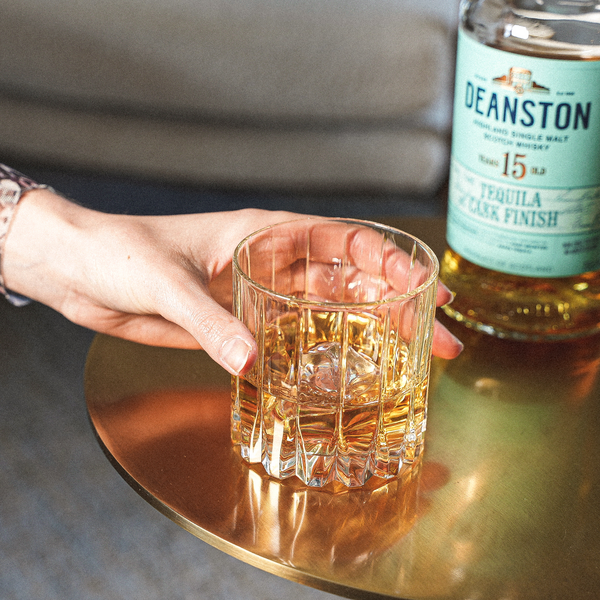In this indoor image, a male hand with a watch reaches for a thick, vertically lined glass of whiskey sitting on a circular gold table. The glass, noted for its ornate, textured bottom, holds a small amount of clear alcohol. To the right of the hand, nestled on the same sophisticated gold table, is a bottle of Deanston Tequila Clark Finish, aged 15 years, adorned with a bluish label. The scene, seemingly promoting this premium alcohol, is set against a backdrop that resembles folded cloth or a couch, enhancing the refined atmosphere.